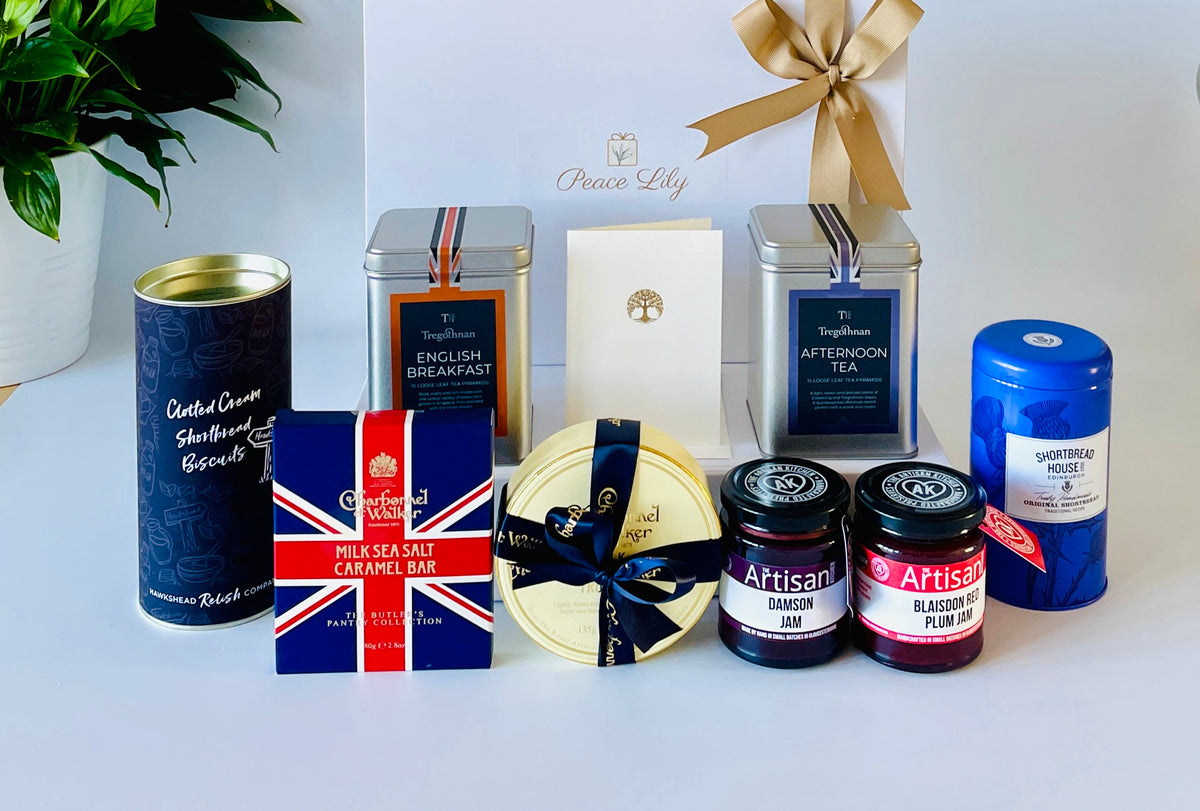The image showcases an elegant display of items typically found in a curated gift basket from Peace Lily. Centered at the back is a sleek gift box adorned with a beige silk ribbon and scripted text reading "Peace Lily," complemented by a logo resembling a gift box. In front of this box, a variety of British-themed gourmet products are meticulously arranged on a white display table. These include two tins of tea—one labeled English Breakfast and the other Afternoon Tea—alongside a tin of Clotted Cream Shortbread Biscuits.

Among the assortment, there is a box of Milk Sea Salt Caramel Bars, decorated with a Union Jack design, lending a distinctly British flair. A round box with a blue ribbon suggests a possible wheel of cheese. Further enhancing the gourmet selection, two jars of artisan jam are presented—one containing Damson Jam and the other Belize and Red Plum Jam, each with labels that sport black print on white backgrounds accented by borders matching the jam's color.

A prominent blue cylindrical tin, inscribed with "Shortbread House," adds to the festive mix of treats. At the forefront, a refined gift card, possibly embossed with a gold bee or flower motif, completes the sophisticated ensemble. The display is enriched by a potted green plant in the corner, likely a Peace Lily, tying back to the brand name and adding a touch of natural elegance to the composition.